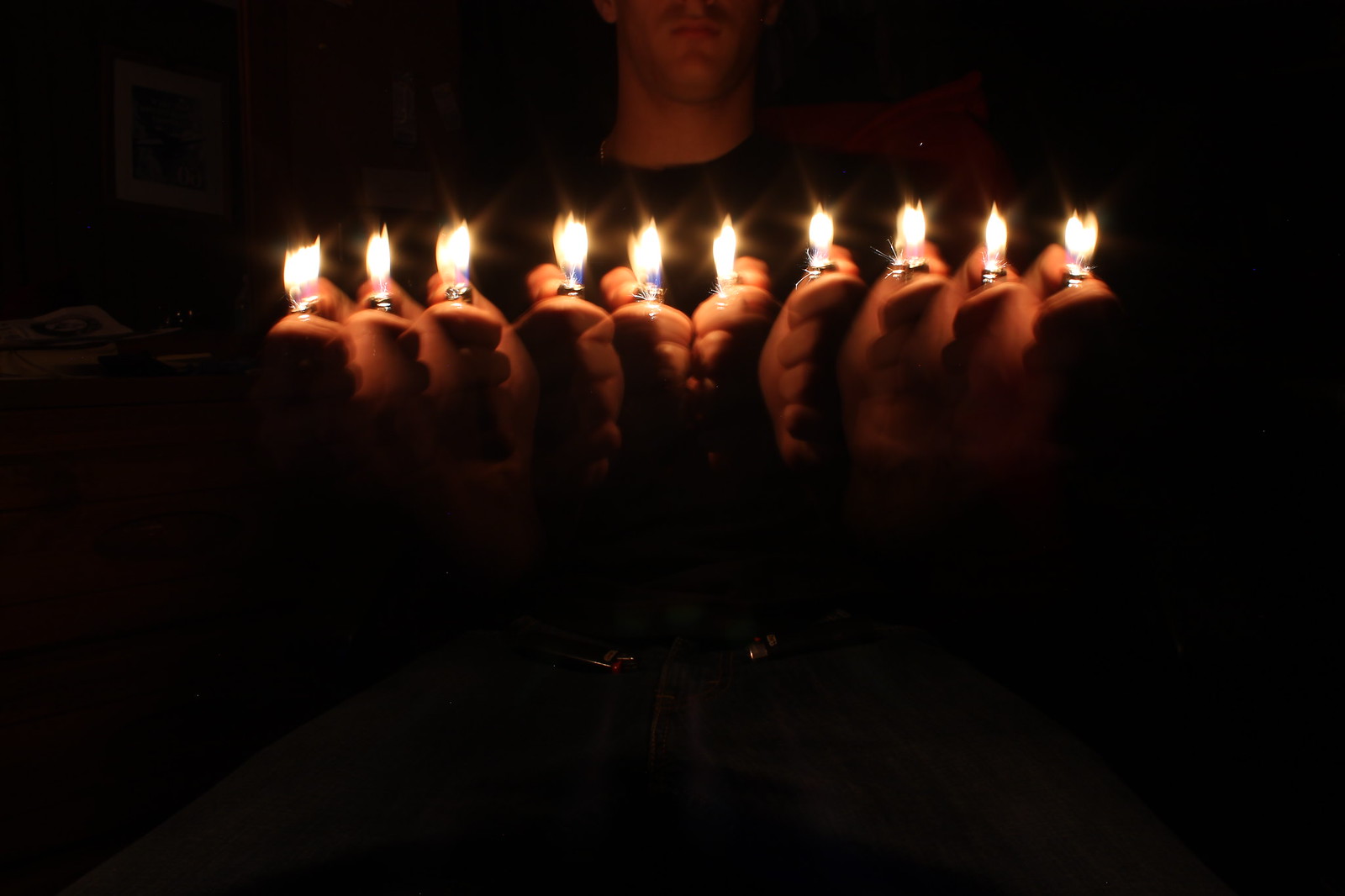A composite photo features the same Caucasian hand multiplied approximately ten times, holding a cigarette lighter in a range of motions. The tightly grouped hands form a line across the middle of the image, with flames above each clenched fist. The person, partially visible from the nose down, has fair skin, a thin mustache, and a dark crew-neck shirt. The background is predominantly black, further emphasizing the hands and flames. Despite slight inconsistencies about visibility of additional objects, the overall effect appears to be achieved through photo editing or creative camera techniques, lending a surreal quality to the image.